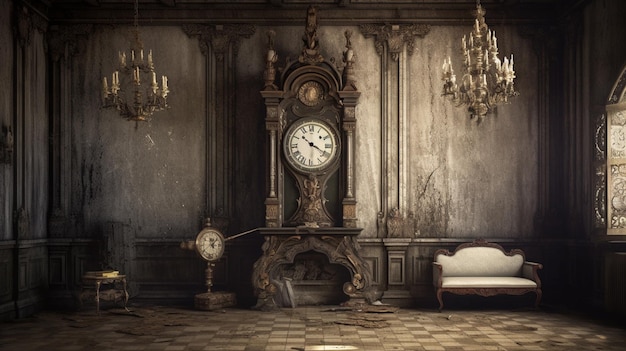The image is reminiscent of a Wes Anderson symmetrical portrait depicting an old Elizabethan or Victorian Age interior. The room, viewed from one side to the other, has dark grey, slightly cracked and molded wallpaper, further accentuated by dark brown, ornate wood carvings and a chair rail along the walls. Centrally positioned is an imposing, built-in grandfather clock adorned with Roman numerals, flanked by large carvings, pillars, and topped by an arch. 

To its right sits an upholstered wooden couch with white cushion seating, while to its left, closer to the wall, stands a brass globe beside a small table. The grandeur of the room is amplified by two chandeliers—one on either side of the clock—each holding multiple candlesticks. The candelabras beside the clock add an antique flair, with the left one featuring two tiers of candles and the one on the right hosting four. The overall ambiance of the room is dark and vintage, with a padded checkered floor that further adds to its historical, time-worn charm.